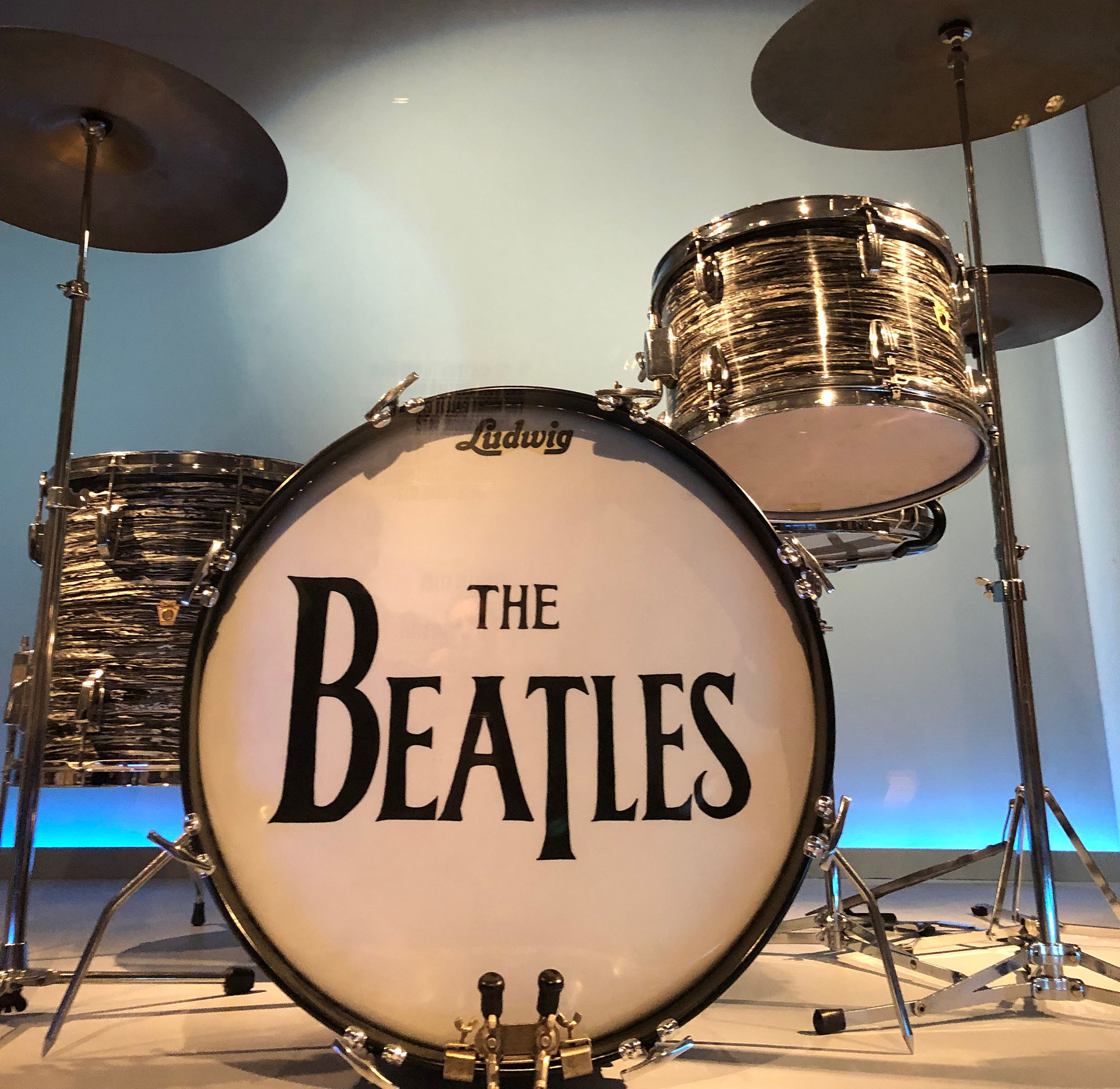The image features a Ludwig drum set adorned with large black letters spelling "The Beatles" on the centerpiece bass drum, which faces directly towards the viewer. The drum kit, shiny and silver, stands prominently on a concrete floor, with a backdrop of white and blue curtains illuminated by subdued lighting, giving a pink, black, gold, and bluish-green hue. The drum set consists of four drums, including an upright tom on the left and a smaller upright drum on the right, partially visible at the bottom. Accompanying these are three cymbals—one above the tom on the left and two to the right, one slightly taller than the other. No performers are present, emphasizing the pristine setup of the iconic instruments, possibly intended for a stage performance, a promotional shoot, or album artwork.